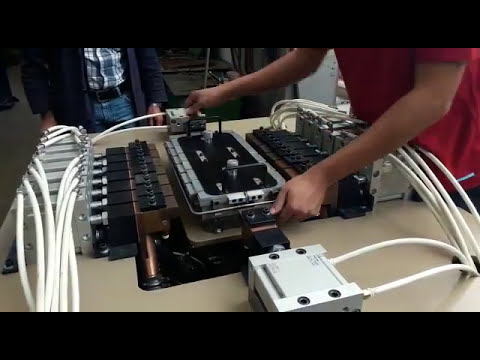In the image, a man in a red short-sleeve shirt is manually manipulating a fuse box or an electrical device, situated in the center of the screen. The device is rectangular with various cables, buttons, and surrounding rectangular components. The cables, predominantly white with metal connectors, extend into a hole on the table. A second man, partly visible in the foreground, is wearing blue jeans, a black belt, a plaid shirt in shades of white, black, or blue, and a black jacket. Both men’s faces are obscured. The surrounding area includes metal shelves and additional wiring. The top and bottom of the image frame are black, adding focus to the busy scene of the hands-on demonstration.